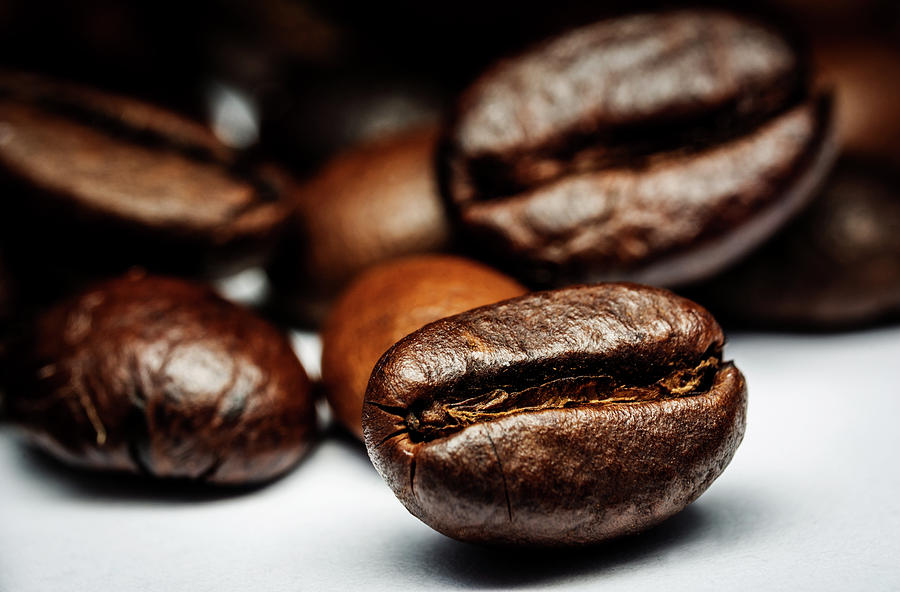The image depicts a white tabletop scattered with coffee beans. Dominating the scene, the coffee beans are predominantly dark brown, oval-shaped, and feature a characteristic central slit. The bean on the right side of the image is particularly in focus, showcasing its detailed texture and coloration, which includes a darker brown exterior and a yellowish hue lining the slit. This bean, reflecting white light, casts a subtle shadow beneath it. In contrast, the beans in the background appear slightly out of focus and vary in color, with some presenting a significantly lighter, mocha brown shade. While most beans rest with their flat sides visible, a few reveal their slits, adding to the visual diversity. The interplay of light and shadow, combined with the varying degrees of focus, creates a rich, textured tableau that emphasizes the unique characteristics of each bean.